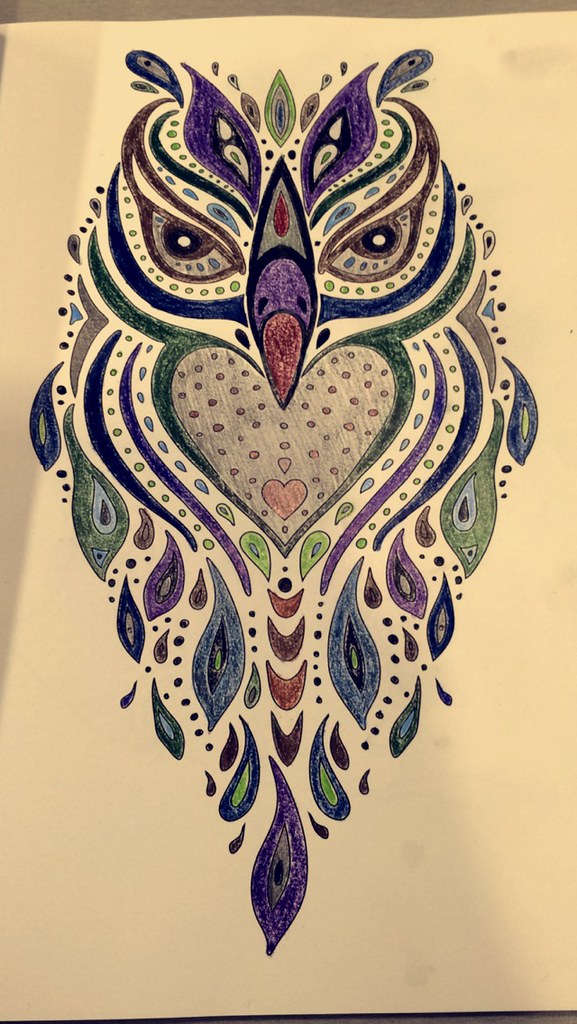The image features an intricate and colorful drawing on a white piece of paper, which appears to be placed on a gray surface. The artwork, predominantly bright and vibrant, depicts an abstract owl with a variety of flowing designs and curvy lines that form its elaborate feathers and body. The owl’s feathers are rendered in teardrop-like shapes, featuring a rich blend of colors such as purple, blue, green, dark pink, and black. The owl’s eyes are large, angled, and brown with white pupils, accompanied by brown eyebrows. At the center of the drawing, there's a prominent heart symbol shaded in grey and pink, with a series of smaller hearts cascading downwards. The beak of the owl is striking with shades of purple, red, and blue, adding to the artistic nature of the piece. Some areas of the paper show gray smudges, enhancing the textured appearance of the drawing. The entire composition captures the essence of abstract artistry, infusing the image with a sense of whimsy and imagination.